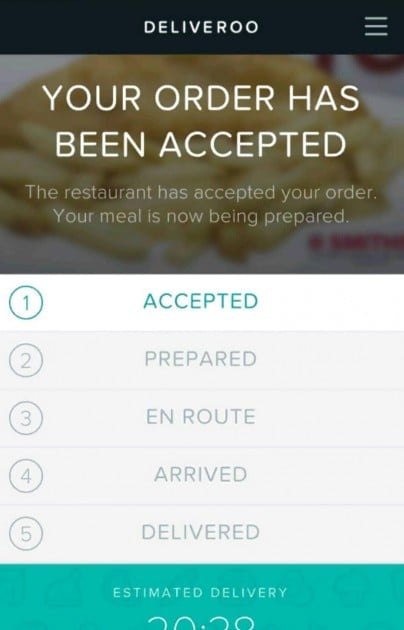In the image captured on a smartphone, the Deliveroo app interface is prominently displayed. At the top, a black rectangle contains the Deliveroo logo, spelled out as "D-E-L-I-V-E-R-O-O." To the right of the logo, there are three horizontal lines indicating a menu that can be clicked. Below this section, the screen displays an announcement in bold, white capital letters stating, "YOUR ORDER HAS BEEN ACCEPTED," with subtext confirming, "The restaurant has accepted your order. Your meal is now being prepared." 

A blurred background image showcasing French fries serves as a backdrop to this notification. Further down the screen, five sequential steps indicating the order process are listed: "1. Accepted," "2. Prepared," "3. Enroute," "4. Arrived," and "5. Delivered." The "Accepted" step is highlighted in teal, while the steps from "Prepared" to "Delivered" are presented in a muted gray.

At the bottom, the estimated delivery time appears in a teal section, although it is partially cut off, reading approximately "20 minutes and 38 seconds."